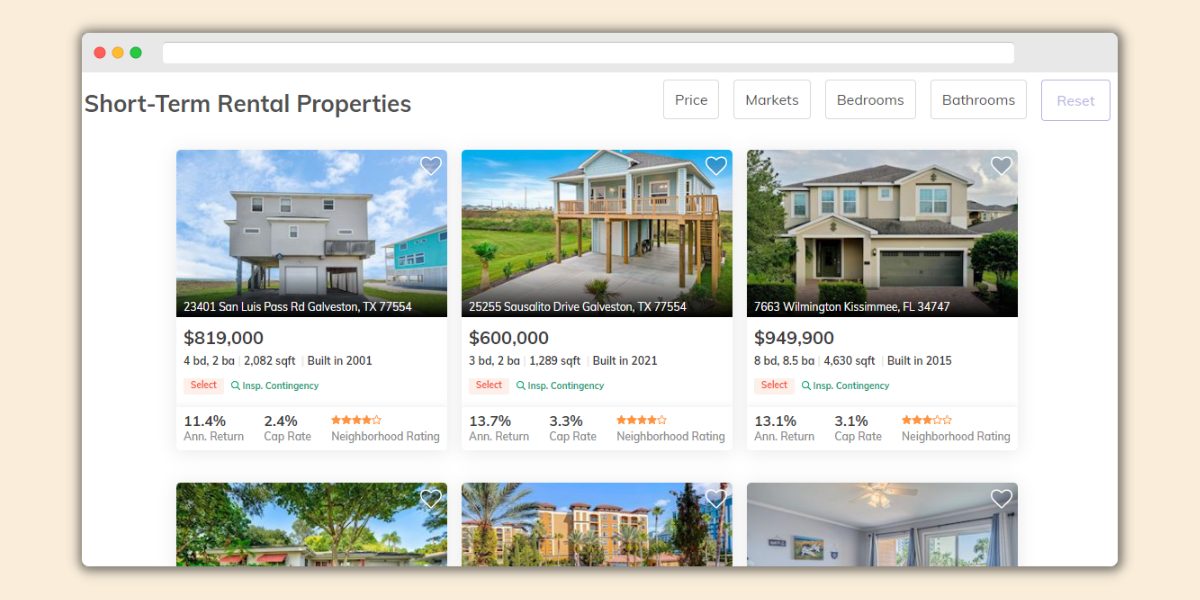A PC screenshot displays a property search webpage for short-term rental properties. The site features a clean, white background with black or dark gray text. At the top left of the screen, the label "Short-term Rental Properties" is prominently displayed. In the upper right corner, there are selectable buttons for filtering results by price, markets, bedrooms, and bathrooms, alongside a 'reset' button for clearing filters. These buttons are subtly labeled against the white background.

Below the filtering options, there are thumbnail previews of six properties, arranged in two rows of three. However, only the top row is fully visible, while the bottom row is partially truncated. The three visible properties include:

1. A property at 23401 San Luis Pass, Galveston, Texas, 77554, listed at $819K.
2. A property on Sausalito Drive, Galveston, listed at $600K.
3. A property in Kissimmee, Florida, listed at $949K.

The layout is straightforward, providing a simple yet effective interface for browsing short-term rental properties.